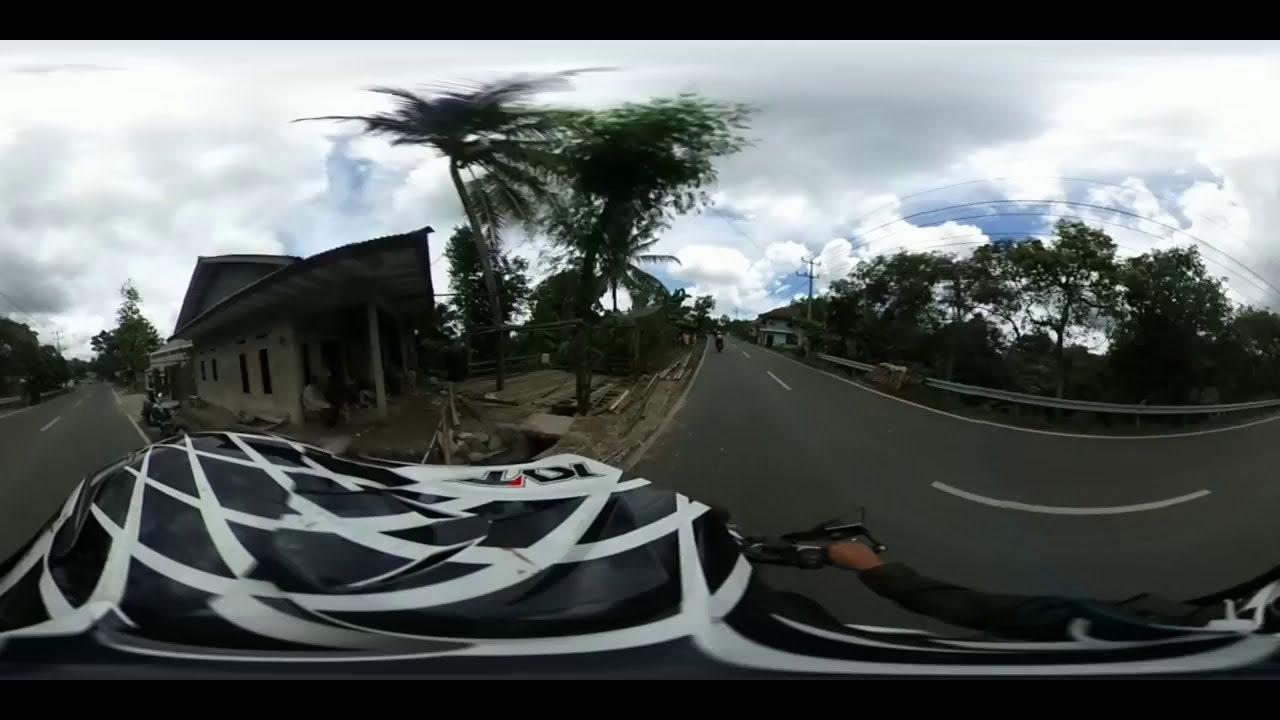This photograph, taken from the rider's point of view on a motorcycle, captures a dynamic outdoor daytime scene with a 360-degree or bubble effect, causing a noticeable distortion. The foreground prominently features the rider’s handlebar and their arm clad in a black long-sleeved shirt, gripping the throttle. Part of the rider's helmet, black with white crisscross patterns, is also visible. 

The road, which appears to be a two-lane one with white lines to the right, stretches ahead. In the distance, another motorcyclist can be seen. On the left side of the road, there's a house or building made of stone, juxtaposed with several palm trees, indicating a warm country. On the right, a metal guardrail runs parallel to the road, with numerous other trees and power lines behind it. 

The sky is predominantly blue with thick, white clouds, suggesting an overcast yet partly sunny day. A narrow black header and footer frame the photograph, enhancing the overall composition and effects applied.